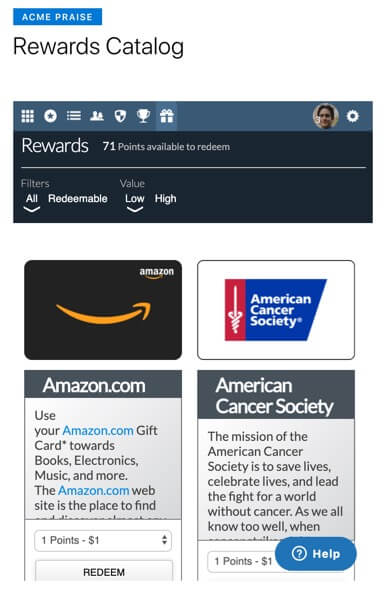This detailed digital screenshot displays the "Acme Praise Rewards Catalog" at the top, indicating that the user has 71 points available for redemption. The profile picture featured in the upper section portrays a young man approximately 34 years old, with a medium skin tone, dark hair, and a cheerful smile.

The forefront of the screenshot prominently showcases a digital image of an Amazon.com gift card, which is stylized in black and orange. Accompanying text explains the versatile usage of the gift card, highlighting its applicability towards purchasing books, electronics, music, and more on the Amazon website. A redeem button is visibly present, signifying that one point is equivalent to one dollar.

Additionally, the screenshot includes the logo of the American Cancer Society, depicted in red, white, and blue, alongside its name. The description of the American Cancer Society's mission elucidates its dedication to saving lives, celebrating lives, and leading the fight for a world without cancer. Lastly, a help button is available for further assistance, reiterating the conversion rate of one point to one dollar.